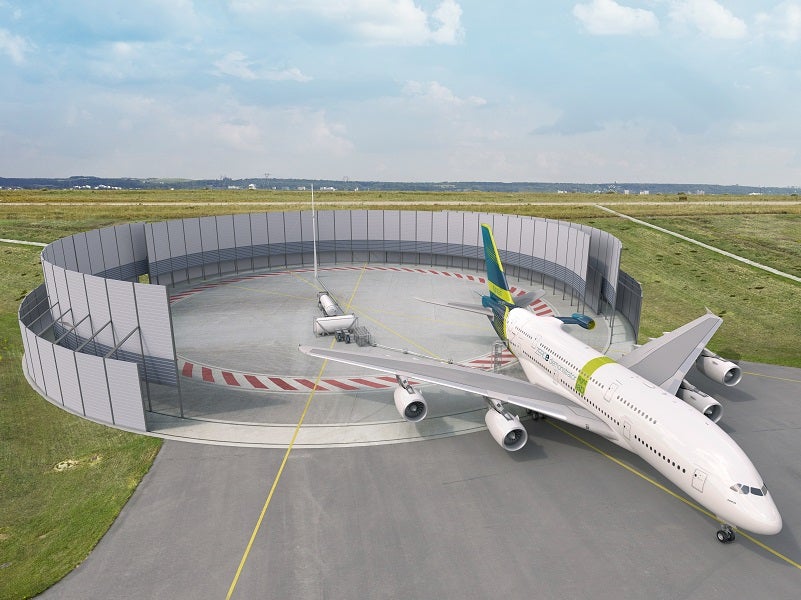In the foreground of the image, a large white passenger airplane adorned with a green horizontal stripe and a teal tail with yellow accents is emerging from a circular barrier area. This circular zone, marked with red and white stripes and a yellow line, appears designed to hold or test aircraft, featuring a protective gray fence shielding it from the surrounding grass patches. The scene extends into a vibrant landscape where green fields transition to yellow at a distance, peppered with distant buildings. Above, a bright blue sky with scattered gray clouds forms a striking backdrop, giving the image depth and a sense of expansive space. The airplane, poised on the runway, looks ready to take flight or move to another location.